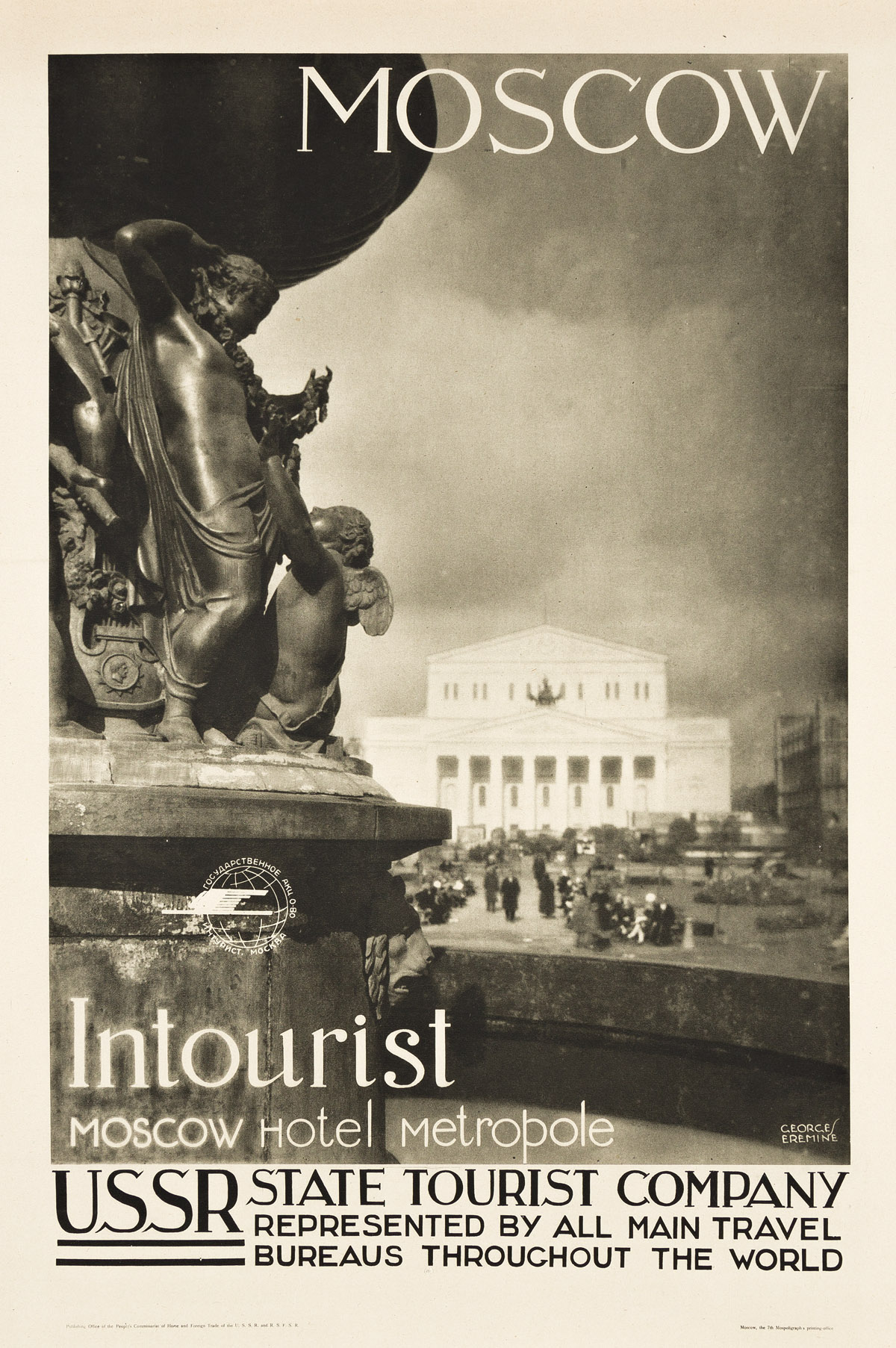This tall, rectangular poster features a muted beige background with "Moscow" prominently displayed in white letters at the top. Below, in off-white writing, it reads, "In Tourist Moscow Hotel Metropole USSR State Tourist Company represented by all main travel bureaus throughout the world." A notable aspect of the poster is a large, pewter-colored statue on the left side, depicting two naked men, one standing and another kneeling, with an emblem and cement base beneath. The statue has a metal-like appearance, consistent with the poster's black-and-white aesthetic. In the background, to the right, stands a white, two-story building, possibly the Moscow Hotel. Scattered in front of the building are blurred, muted figures, giving the scene a bustling yet indistinct look. The name "George Ermine" is inscribed in the far right corner, and a small, barely legible globe is positioned at the bottom. The overall composition, with its detailed depiction of the statue and the architectural backdrop, evokes a sense of historical and cultural significance, despite the cloudy and diffused scene.